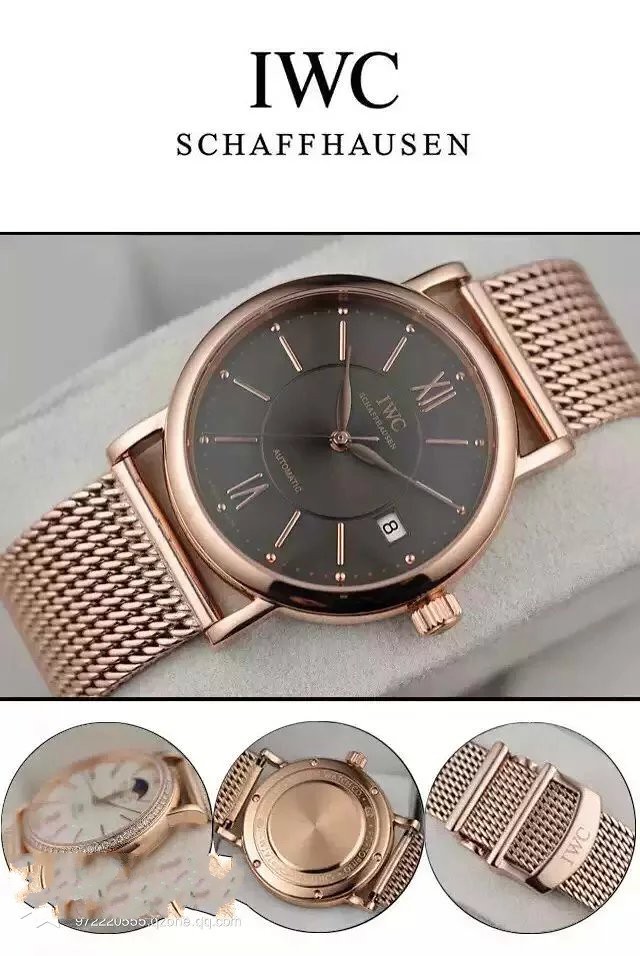This detailed image features a luxurious IWC Schaffhausen watch showcased against a white background with black text reading "IWC Schaffhausen" at the top. The centerpiece is a large, rectangular photograph of the elegant watch, slightly tilted to the right. The watch, which appears to be made of gold with a rose gold hue, boasts a sophisticated design. It has a black face adorned with long, thin, brushed gold hands, and Roman numerals at the 12 and 6 o'clock positions. The other hour markers are represented by seven gold rings. The watch also features a digital display showing the date, specifically the number 8, in black text against a white background. The band is a gold chain-link style, transitioning seamlessly to the watch's circular frame. 

The main image is complemented by three smaller circular insets at the bottom, providing additional perspectives: a top-right angled view, a detailed look at the bottom or backside of the watch, and a close-up of the gold clasp. The composition and detailed presentation of multiple angles make this a comprehensive advertising image, likely intended for a catalog.